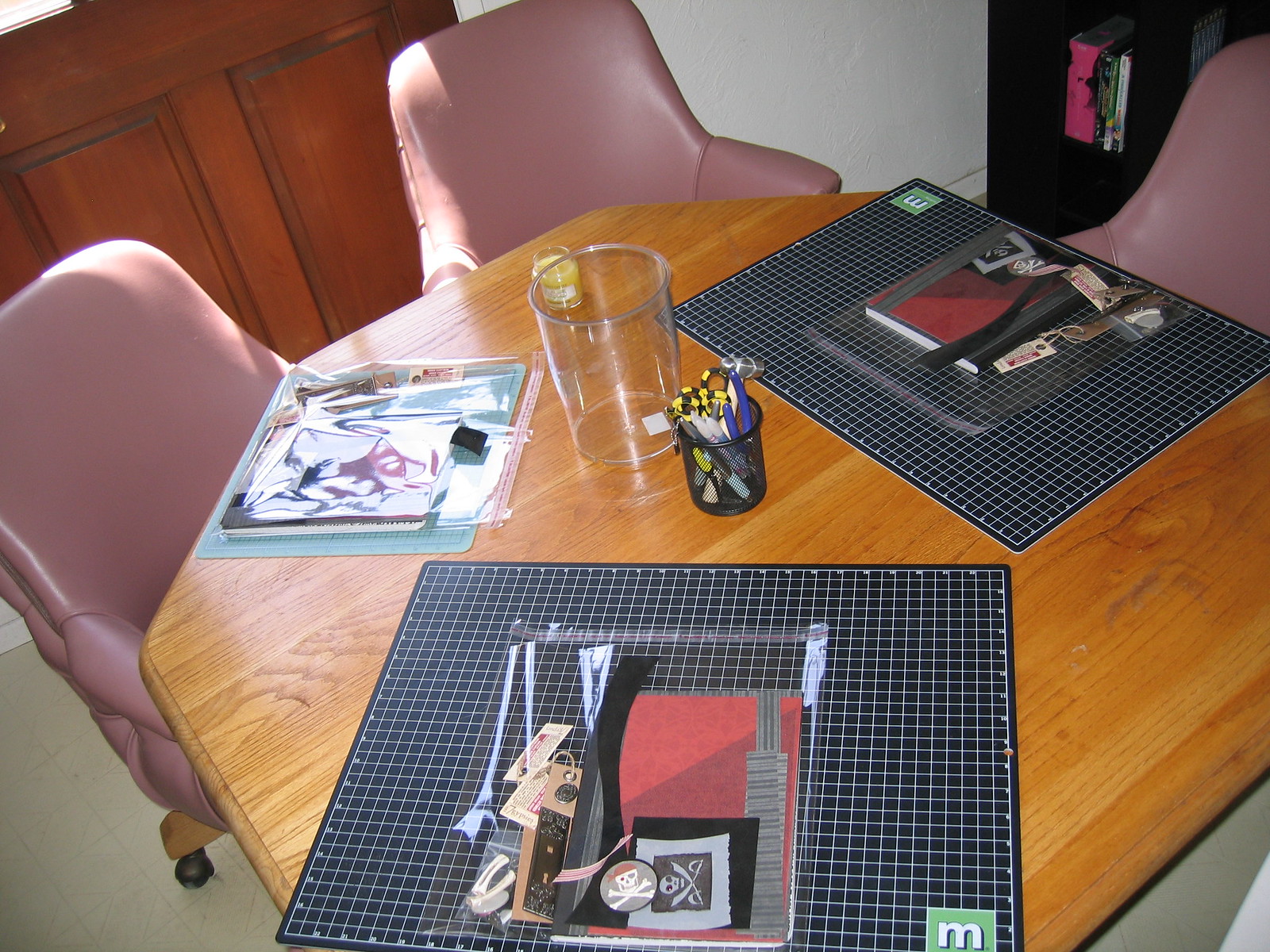This image depicts a cozy corner of a home, possibly a kitchen or dining room, featuring a meticulously detailed scene centered around a wooden octagon-shaped table. The room is adorned with light-colored, off-white to cream tiled flooring, complemented by pristine white walls and baseboards. A darker wooden cabinet stands against the backdrop, accompanied by a black shelf on the right side which holds a few indistinguishable items.

The table itself showcases a light to medium wood finish and is surrounded by chairs with wooden bases on wheels, upholstered in a delicate mauve hue. The surface of the table is an arts and crafts haven, displaying various crafting supplies. Noteworthy among these are cutting mats—two with a black background and white stripes, and a smaller, lighter blue one. Each cutting mat is topped with a plastic bin or ziplock bag brimming with assorted components, perhaps stickers featuring skulls and crossbones, though the exact contents remain unclear. Also present on the table are a notebook, a pencil holder filled with pens, pencils, markers, and pliers, a small candle, and a larger glass.

This detailed vignette captures the essence of a well-used creative space within a warm, inviting home environment.